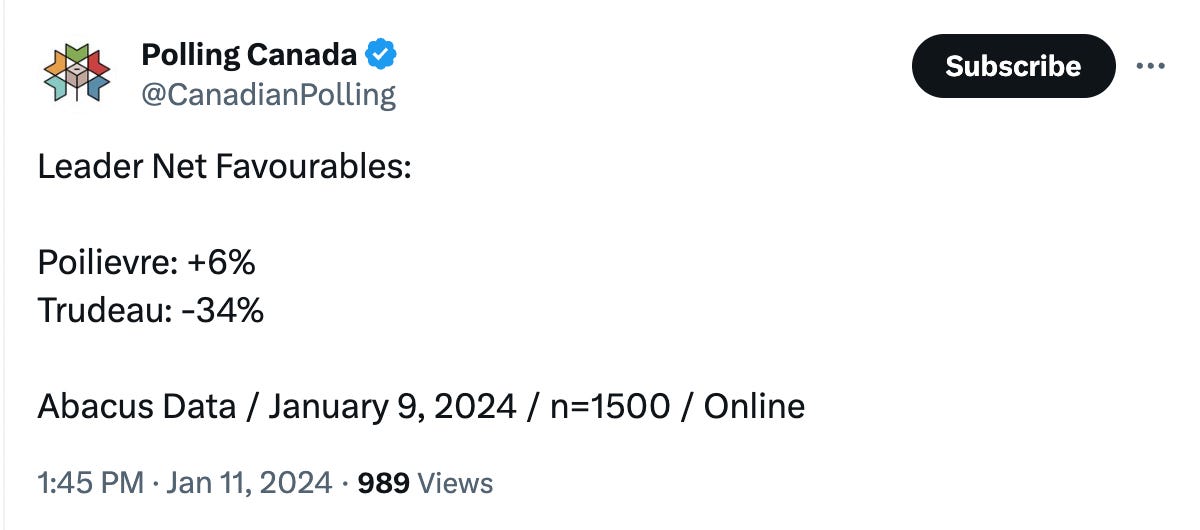The image is a screenshot from an old tweet on the platform now known as X, formerly Twitter. The page features a white background. In the upper left corner, there is a logo resembling a leaf with a grayish-brown cube at its center. Surrounding this cube, starting from the bottom left and curving around, are arrows in various colors: sky blue, orange, green, dark blue, and red.

The account name, "Polling Canada," is displayed alongside a blue check mark, indicating it is a verified account. The tweet contains information about leader net favorabilities, showing "Polly Ever" with +6% and "Trudeau" with -34%.

The data is sourced from "Bacchus Data," dated January 9, 2024, with a sample size (n) of 1,500 respondents, collected online.